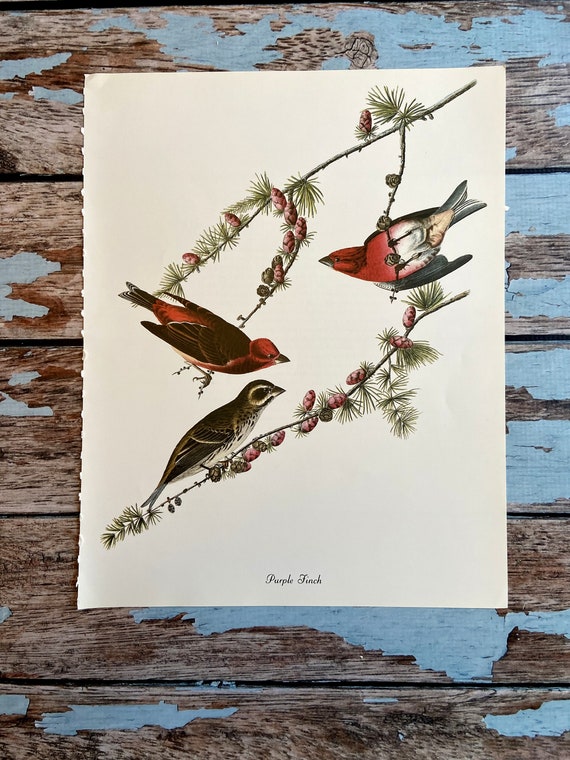The photograph depicts a rectangular sheet of beige paper with a detailed drawing of three birds perched on branches. The sheet of paper has tears and perforations along the left edge, suggesting it was torn from a book. The branches, with thin needle-like leaves and small, brown, pinecone-shaped seeds, stretch from the right side of the paper towards the left. Two birds are depicted on the upper branch, while one bird is on the lower branch. The bird on the right is red and white, the upper bird on the left is red and black, and the lower bird is black and white. At the bottom of the paper, the text "Purple Finch" is printed in a cursive font. The paper is placed on a flat wooden surface that was once painted blue, but the paint is chipped, revealing the bare wood underneath. The wood has horizontal slats, with some areas appearing dark brown.